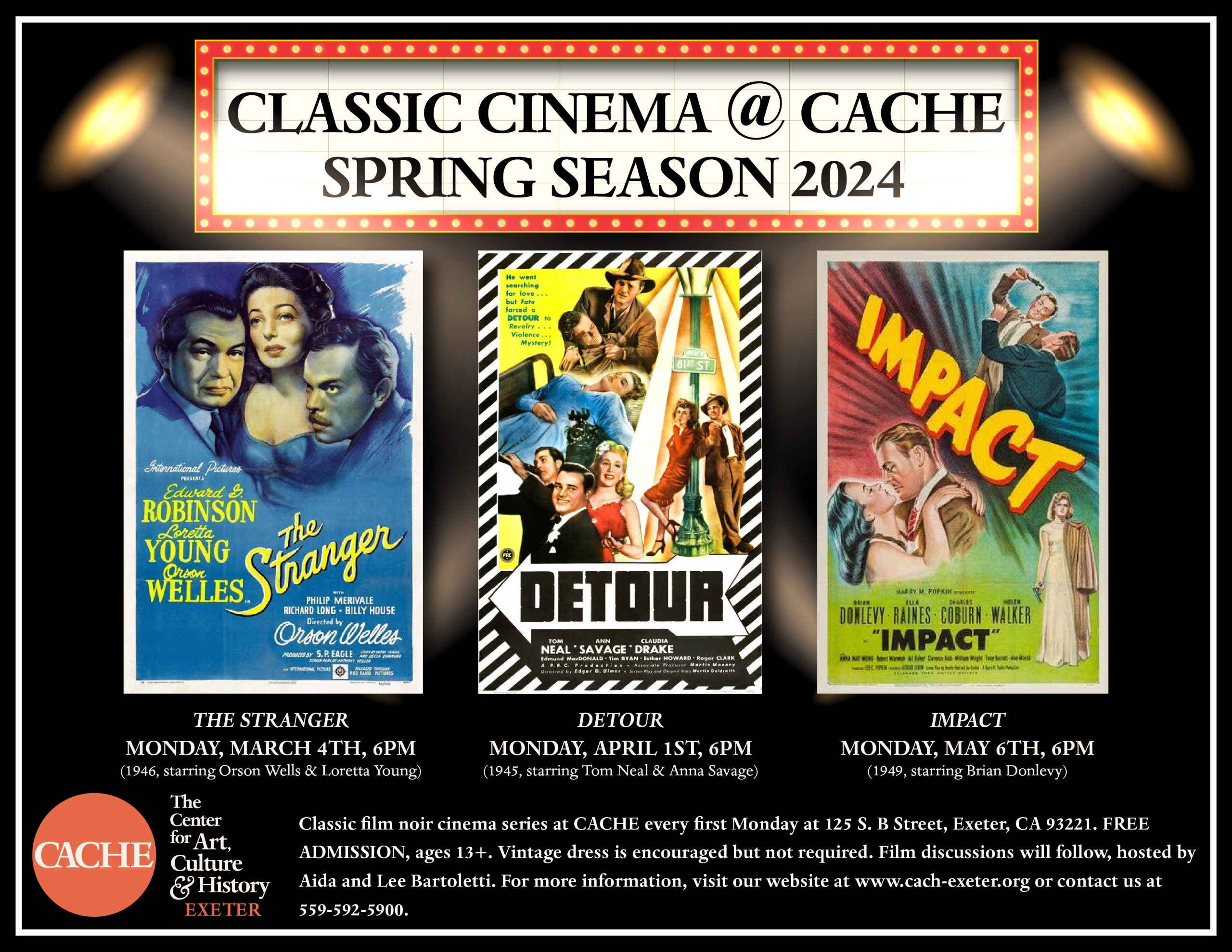The image is a landscape-oriented poster for an event at the Center for Art, Culture, and History Exeter (C-A-C-H-E). The top section features a bold, movie billboard-style header outlined in orange with white dots, which reads "Classic Cinema at C-A-C-H-E Spring Season 2024" in two lines of black text. To either side of this header are spotlights casting rays diagonally downward—one from the left and one from the right.

Beneath the header are three vintage-styled movie posters:
1. The left poster, titled "The Stranger," prominently displays the title in yellow letters on the right side and features the faces of three actors—two men and one woman—situated at the top. The names of the actors are listed on the left, all set against a blue-hued background.
2. The middle poster, titled "Detour," showcases various colorful illustrations of characters and scenes from the movie, such as dramatic moments and iconic encounters, with the title in large black letters across the bottom.
3. The right poster, entitled "Impact," has its title in striking yellow letters diagonally from the upper left. It depicts a man about to strike another man in the top right corner, and a couple about to kiss in the bottom left. Actor names are provided at the bottom in black text.

At the footer of the poster, beneath each movie display, are dates and times for the screenings, along with additional small white text details. The bottom left-hand corner features an orange circle logo with "C-A-C-H-E" in white, next to the name "Center for Art, Culture, and History Exeter," and further information in small orange and white text.